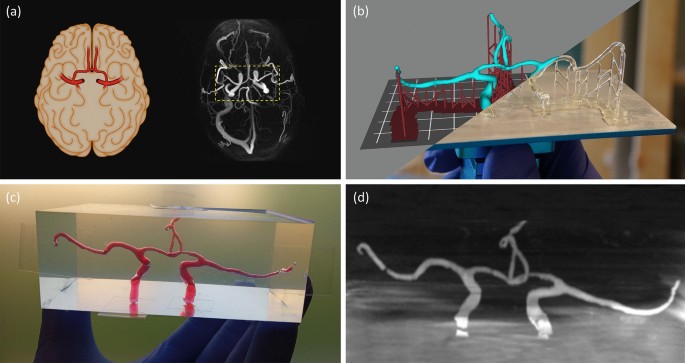The image is a composition of four equal-sized rectangular pictures labeled A, B, C, and D. 

Top left (A) features a black background with a stylized illustration of a brain in tan, highlighted by brown lines and red areas that resemble veins. Adjacent to it is a black-and-white x-ray of a brain lit up. 

Top right (B) showcases a grayscale background with a side-by-side comparison: to the left, a color drawing of a bridge in red and green, and to the right, a color photograph of the bridge, seemingly constructed from toothpicks.

Bottom left (C) shows a blue-gloved hand holding up a transparent, rectangular lucite box encasing red, intricately squiggly shapes.

Bottom right (D) presents the same red squiggly shapes in a black-and-white photograph, mirroring the contents of the lucite box shown in image C.